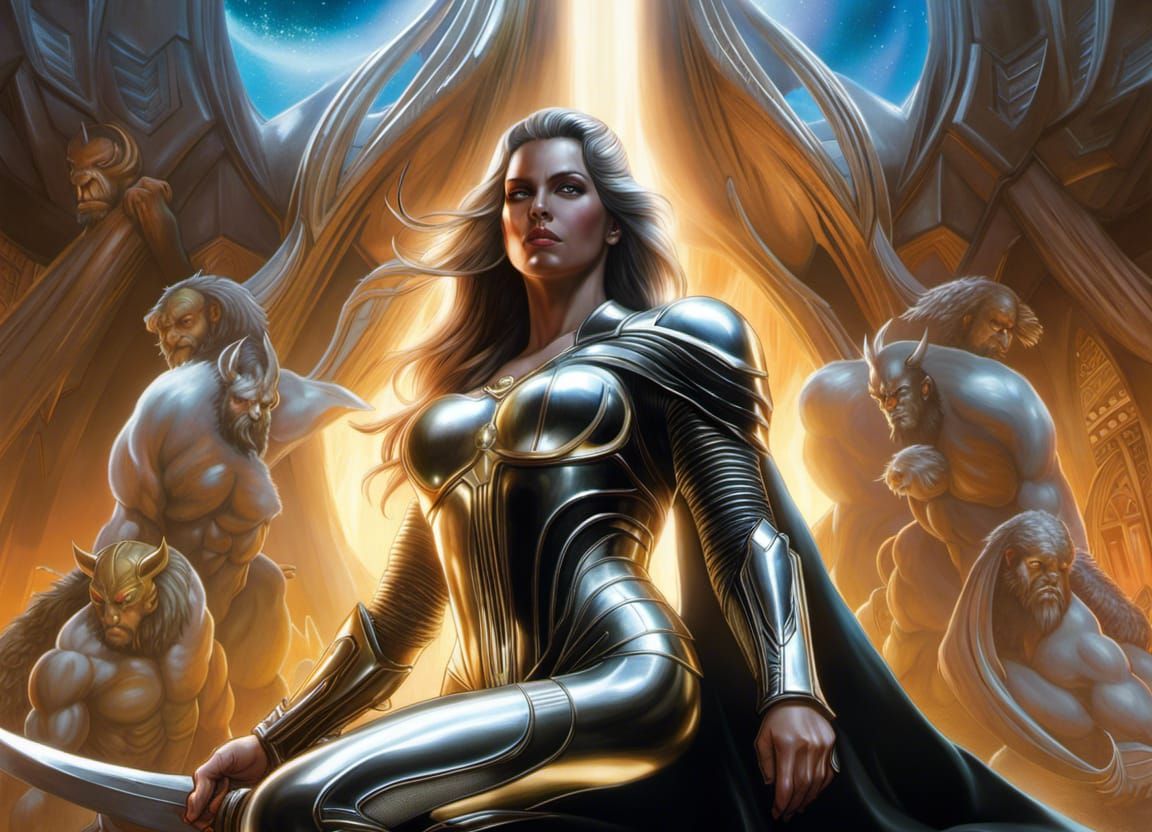The image depicts a scene that appears to be from a sci-fi or fantasy genre, likely computer-generated or a detailed artwork. At the center is a striking female character with long, flowing blonde hair, partially captured in a semi-profile view. She wears an elaborate suit of shiny silver armor adorned with gold trim and sports a black cape. The woman is holding a large dagger or sword in her right hand and stands with an upright, intense posture, suggesting readiness for combat.

Surrounding her on both sides are several fantastical, muscular creatures that appear to be hybrids of humans and animals, each with horned or masked faces. These creatures are depicted using hues of gold, browns, and sepia tones, giving them an almost demonic or mythical appearance. Some resemble devils with golden horns, while others have gorilla-like faces or are covered in fur.

The background features an ornate, temple-like structure, and through an opening at the top, a bluish-white nighttime sky is visible. A dramatic beam of glowing gold or orange light cascades down from above, creating a radiant aura around the main character. The overall scene suggests a setting of significant importance, perhaps within a large building or ship, and emphasizes the central figure as a powerful, combat-ready protagonist amidst a host of formidable creatures.